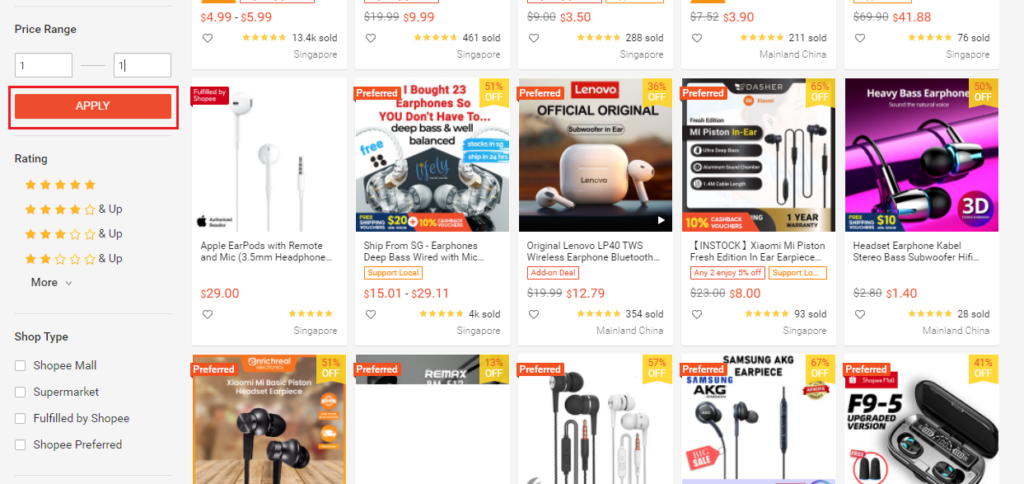This image is a screenshot from an e-commerce website showcasing a variety of audio products. In the upper left-hand corner, there's a search feature allowing users to specify a price range, with a default set at $121. Below this, a red "Apply" button in white lettering can be clicked to filter the results based on the specified price range. To the side, a ratings system displays options for 5-star, 4-star, 3-star, and 2-star products. The image also shows category filters such as Shop Type (Shoppy Mall, Supermarket, Fulfilled by Shoppy, and Shoppy Preferred).

The main section of the image reveals a grid layout with two rows of products, each containing five items. The top row includes:
1. Apple EarPods with remote and mic.
2. Deep Brass Wired Microphone.
3. Wireless Bluetooth Earphone.
4. Exome Piston Fresh Edition Earpiece.
5. Stereo Bass Subwoofer Hi-Fi Earbuds.

The bottom row similarly features a variety of earphones, both AirPods and wired earbuds, highlighting the focus on personal audio devices. Each item is visually represented with clear images, showcasing the diverse range of listening options available for purchase.